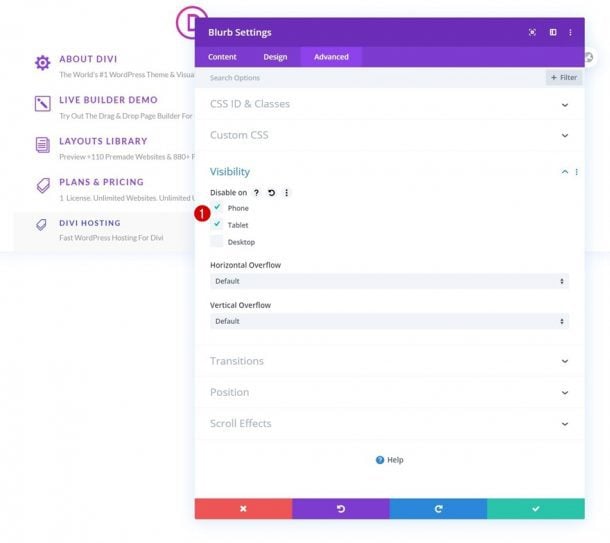This is a screenshot of a theme building page. On the left side, there are various menu options displayed in purple font. Adjacent to these options is a widget icon. Below it, the text reads "Divi, the world's number one WordPress theme and visual," but the sentence is incomplete. The following line contains a square icon with a pencil in its center alongside the text "Live Builder Demo - Try out the drag-and-drop page builder," although this line is also partially truncated.

Further down, there is an icon resembling a sheet of notebook paper, next to the text "Layouts Library - Preview over 110 pre-made websites." Another item features a tag icon and the text "Plans and Pricing - One license, unlimited websites." A second tag icon follows with the text "Divi Hosting - Fast WordPress hosting for Divi."

On the right side of the screen, an overlaid image displays a page with a purple banner at the top, followed by a lighter purple banner beneath it. The bottom section of this page contains four distinct rectangular sections colored in orange, purple, blue, and green.